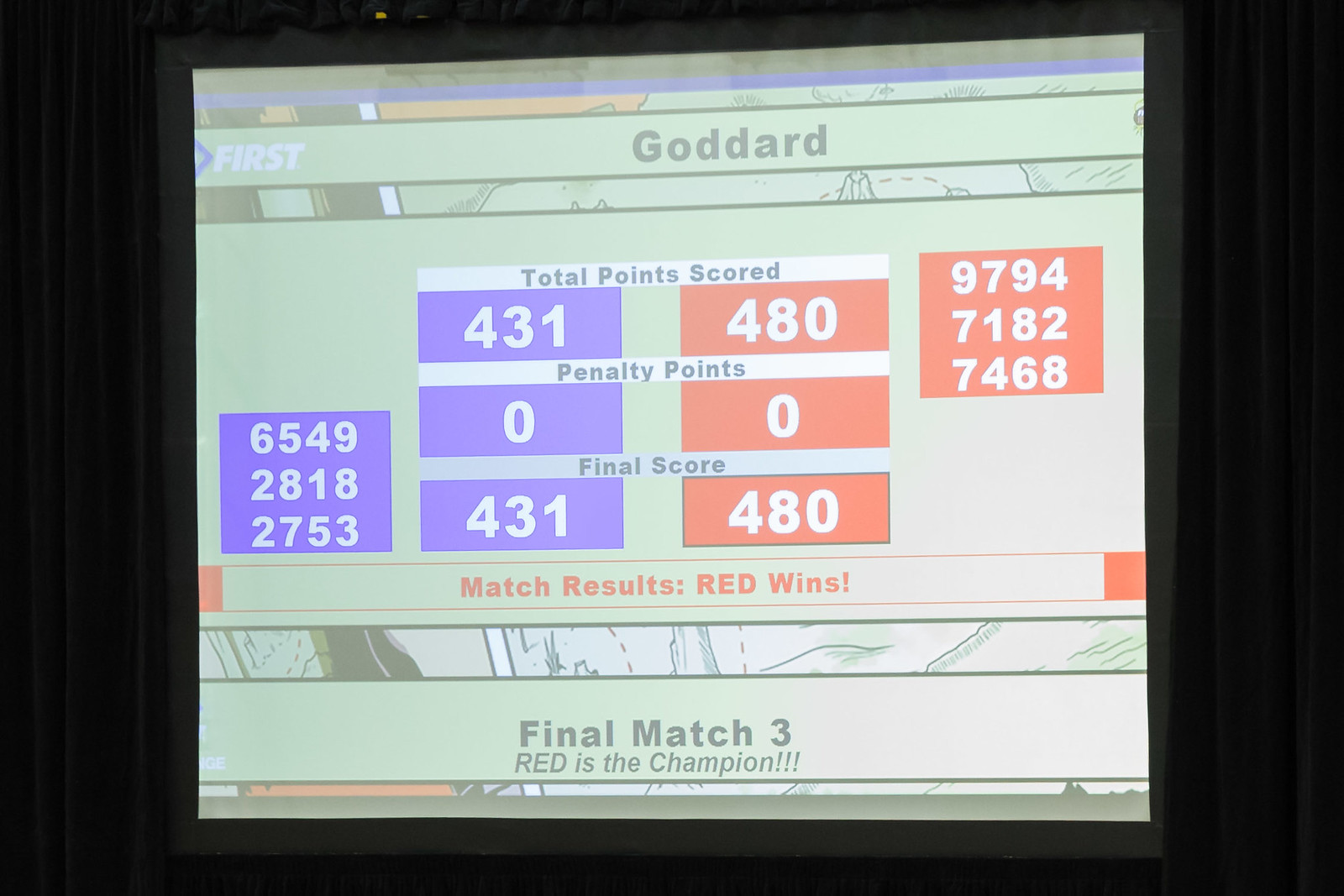This photograph, taken of a screen, displays detailed information regarding a competitive match. At the top of the screen, it reads "First Goddard," with two columns below – one blue and one red. The first row lists "Total Points Scored" with 431 for blue and 480 for red, followed by "Penalty Points," showing zero for both teams. The "Final Score" row reiterates 431 for blue and 480 for red. Beneath, in red text, it declares "Match Results: Red Wins," and further below, it announces in black text, "Final Match Three: Red is the Champion!!!" On either side of the chart, additional numbers are displayed within red and blue boxes, but their specific function is unclear. The background of the image appears drawn but remains indiscernible. The scoreboard has a striking contrast against a black backdrop, with blue and red color coding highlighting the respective teams.